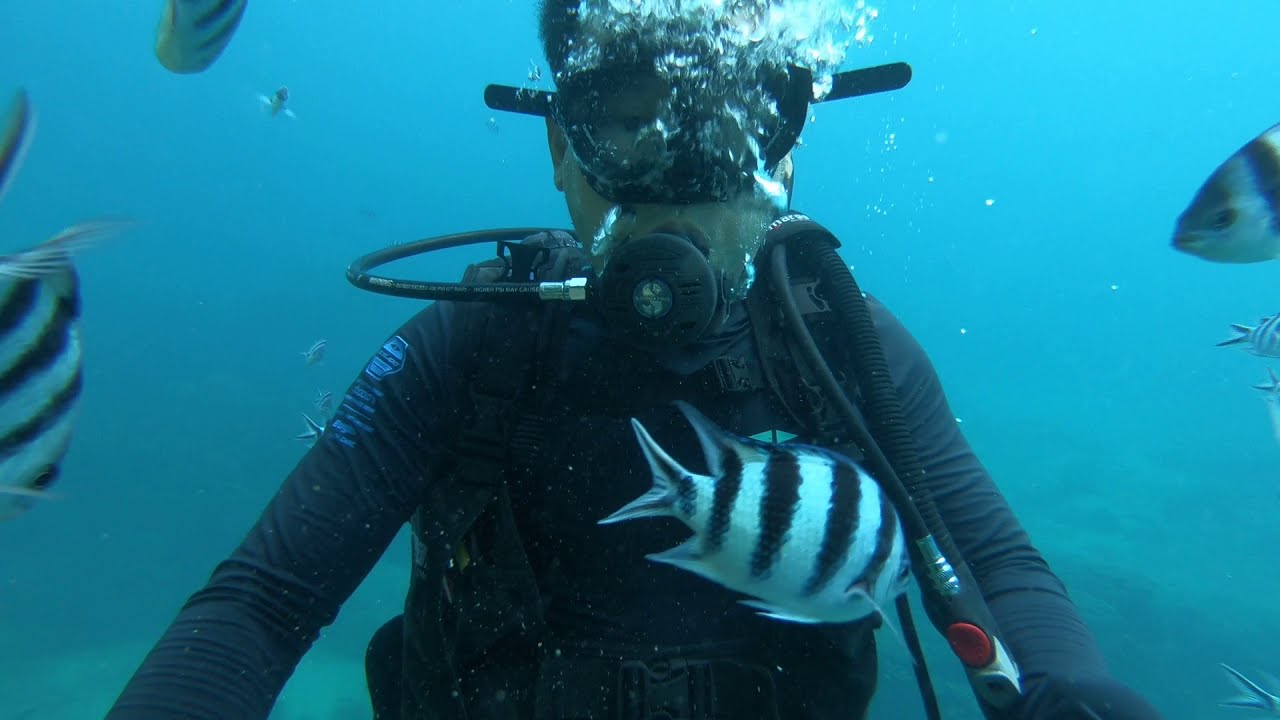An underwater photograph captures a scuba diver in the ocean, framed from the waist up and centered in the image, set against a backdrop of crystal clear, turquoise waters. The diver is dressed in a black wetsuit, featuring a logo on the left arm, and equipped with black goggles and a large mouthpiece connected to a long hose that wraps around his body, with a noticeable red button on it. A multitude of bubbles rise from the diver's mouthpiece, partially obscuring his masked face and head. Around the diver, a group of five black and white striped fish swim prominently in the foreground, with additional similar fish blurred in the background, adding lively detail and motion to the serene aquatic setting.